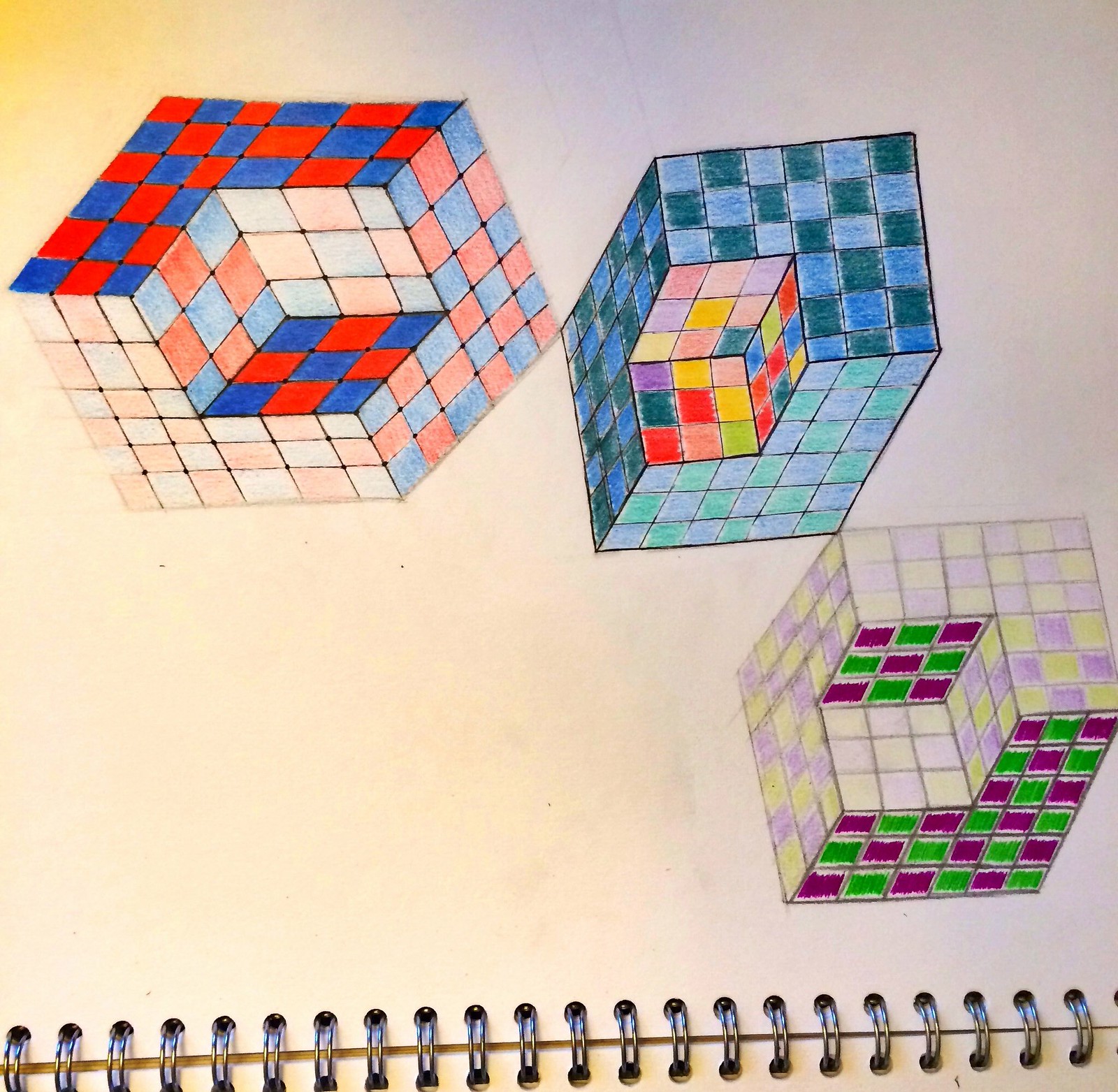This intricate drawing on notebook paper features three three-dimensional Rubik's Cubes, meticulously colored with colored pencils. The notebook is oriented horizontally, with the spine located at the bottom of the image. The first Rubik's Cube is positioned near the bottom right corner, displaying a mix of green, pink, and yellow hues, with some sections appearing slightly faded. Directly above this cube is a second one, vibrantly illustrated in a variety of colors including orange, yellow, purple, and blue. To the left of this middle cube is the third Rubik's Cube, showcasing a predominantly orange and blue color scheme. All three cubes are crafted with attention to detail, making the drawing both dynamic and visually engaging.